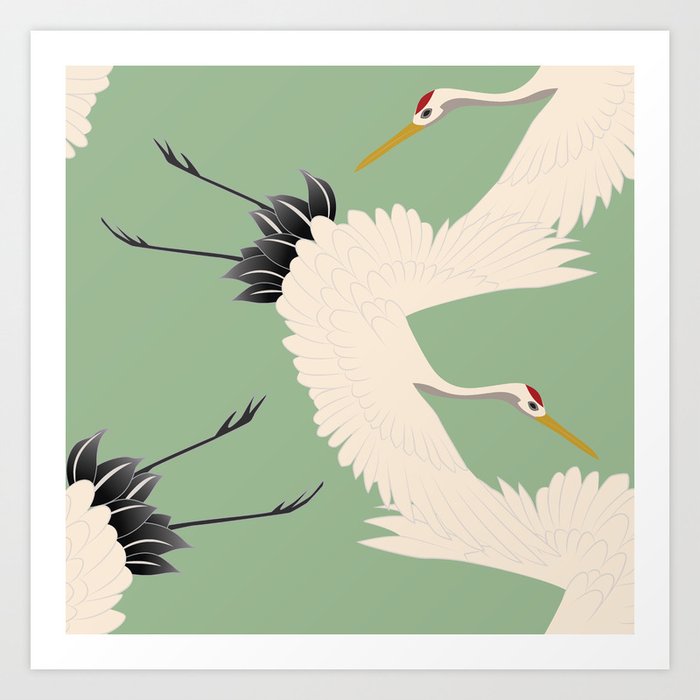The image depicts a detailed, stylized painting of several cranes with a sage green background. The centerpiece of the image is a crane with distinctive features: a long gold beak, a small head with a red spot on top, a black eye, white feathers, black tail feathers, and long, thin black legs. Surrounding this main crane, there are glimpses of additional cranes; one is visible only by its head and one wing in the top right corner, another shows just its legs, and a final bird reveals a partial wing. These cranes appear to be flying in various directions, creating a dynamic composition. The painting is framed with a white matte and complemented by a secondary gray frame, enhancing the overall presentation. The crisp and sharp edges of the birds contrast with the soft, fluffy texture of their feathers, making the illustration both vivid and detailed.